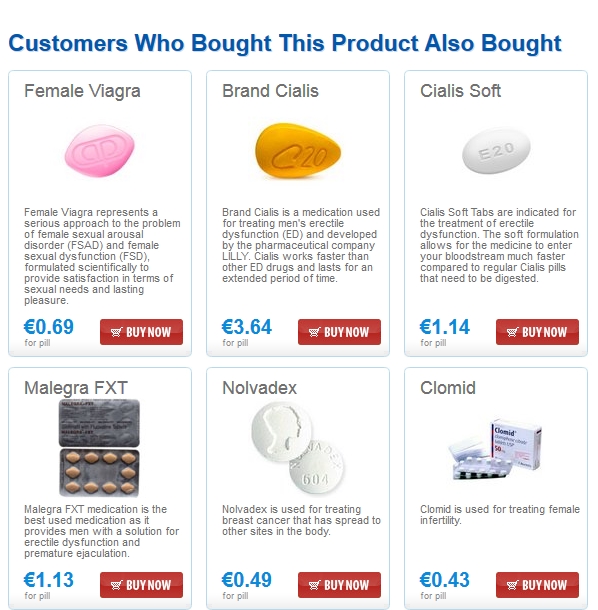At the very top of the image, written in blue text, it states, "Customers who bought this product also bought."

First Row (Left to Right):
1. In the first square, there is an item labeled "Female Viagra," represented by a pink pill. Below it, the price is listed in blue as $0.69 per pill. Underneath the price is a red rectangle featuring an image of a shopping cart and the words "Buy Now."
2. To the right is "Brand CIALIS," depicted as an orange pill with "C-20" printed on it. The price is $3.64 per pill, and there is an option to "Buy Now."
3. The third item is "Cialis Soft," illustrated as a white pill with "E-20" printed on it. Below this, the price is $1.14 per pill.

Second Row (Left to Right):
1. On the left, the item "Malagra FXT" is displayed, priced at $1.13 per pill. The image shows several orange oval-shaped pills inside a container.
2. To the right of this is "Nolvadex," represented by two white pills. The price is $0.49 per pill.
3. Finally, there is "Clomid," shown as a box of pills, with a price of $0.43 per pill.